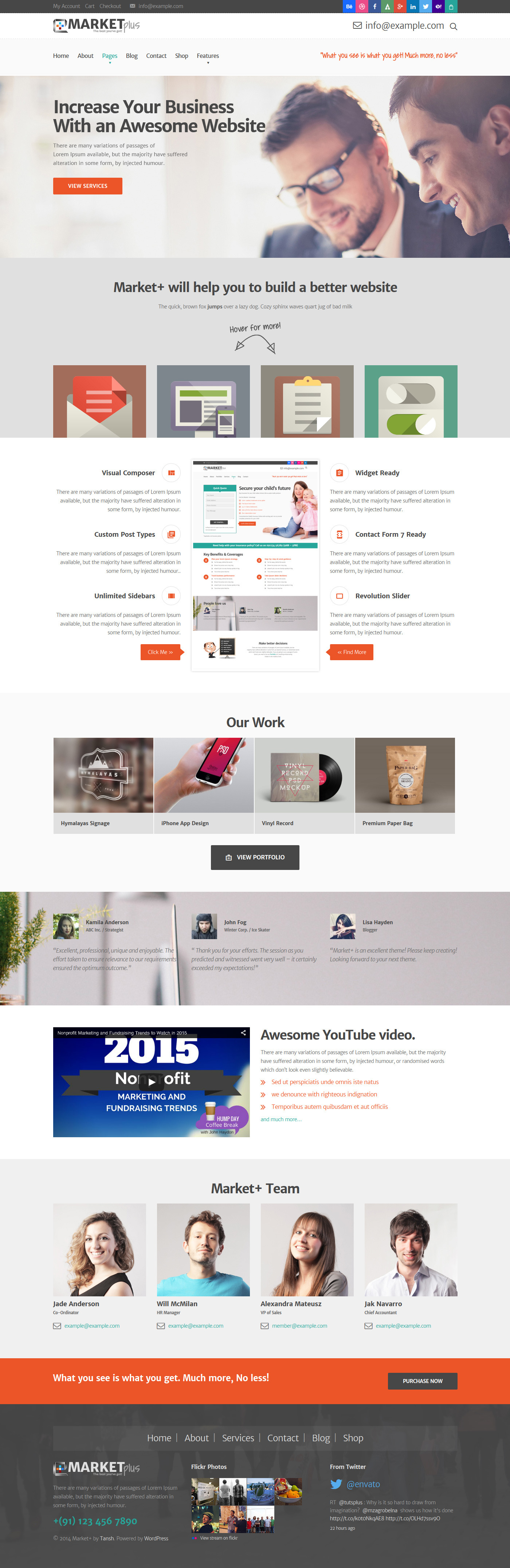Screenshot of an e-commerce website showing a detailed layout. 

At the top, there is a black navigation bar containing multiple social media icons. Directly below this bar, in bold black text, is the word "Market." Beneath the header, there's a list of small options accompanied by orange text. 

The primary visual element is an image of two men, both smiling; one man has glasses and short hair, while the other has short hair and no glasses. Overlaid on the image is a text that reads, "Increase your business with an awesome website." Below this, there is a brief paragraph followed by an orange call-to-action button.

Further down, a black heading states, "Market will help you to build a better website." Adjacent to the text are four images.

Continuing, there are three small pictures, including one of a woman and a small child. Below these images, a black text heading reads, "Our Work," followed by four additional small images displaying various items, including a glass, a shop window, a phone in someone's hand, a record, and a bag of groceries.

At the very bottom, there are images labeled "Market and Team," featuring four different people.